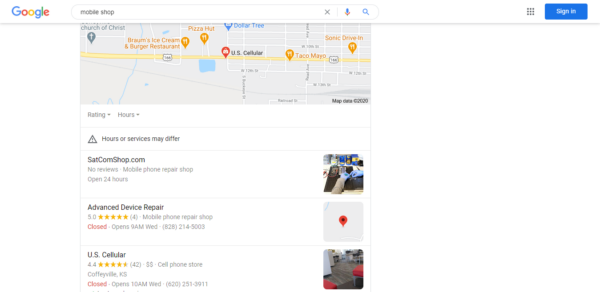The image is a detailed screenshot of a Google Maps search result for "mobile shop." In the upper left corner, the search bar displays the query "mobile shop." The map highlights various nearby locations including Sonic Drive-In, Taco Mayo, US Cellular, Pizza Hut, and Brahms Ice Cream and Burger Restaurant. A note mentions, "hours or services may differ."

On the left side of the image, there is a listing for "satcomshop.com," described as a mobile phone repair shop with no reviews, open 24 hours. To the right of this, a grainy photograph shows a pair of hands, clad in blue gloves, meticulously repairing a computer.

Below, there is an entry for "Advanced Device Repair," noted as a five-star mobile phone repair shop with four reviews. It's indicated that the shop is closed and will open at 9 a.m. on Wednesday. Additionally, US Cellular is listed with 828 reviews, 4.4-star rating, and 42 reviews specific to a section marked with two dollar signs, indicating it is a moderately priced cell phone store.